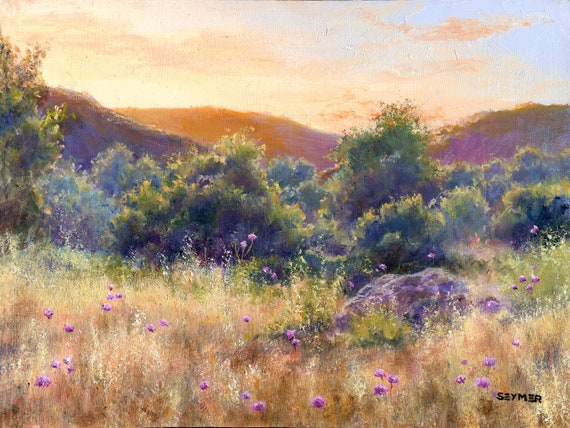This richly detailed oil painting captures an enchanting springtime outdoor landscape at sunset. The foreground features a meadow interspersed with vibrant purple wildflowers blooming amidst orangey-gold tall grass. A modest rock can also be seen among the flowers, adding texture to the scene. Just behind the meadow, a row of tall bushes and trees lead the eye toward the horizon, where rolling hills and modest mountains, perhaps 200 to 300 meters high, glow warmly under the radiant sunset sky. The sky itself is a mesmerizing blend of orange and yellow hues, with patches of blue still visible, and is adorned with beautifully rendered clouds. No human presence or man-made objects detract from the natural beauty depicted. The painter's name, "Seymer," is elegantly signed in text at the bottom right corner of this serene and evocative landscape.